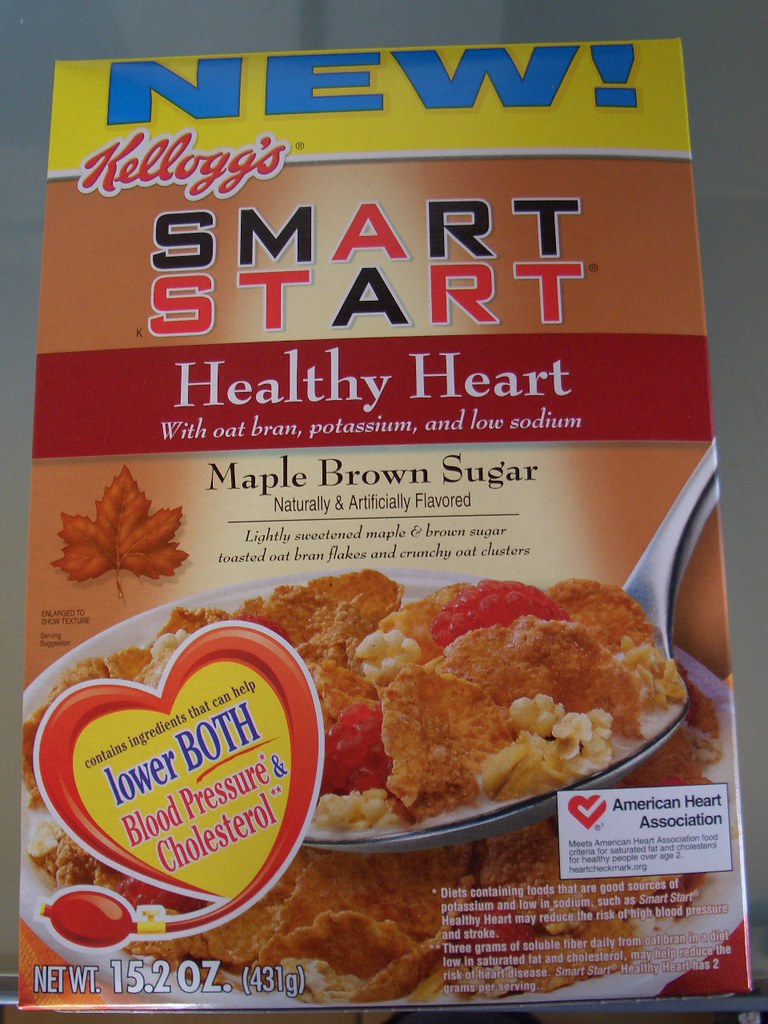This photograph features a cereal box placed against a grayish background with a metallic edge, suggesting it might be set on a table. The cereal box prominently displays the word "NEW" in large blue letters on a yellow background. The brand name "Kellogg's" appears in the standard Kellogg's font. The cereal's name is "Smart Start" written in alternating black and red fonts. 

Beneath this, the tagline "Healthy Heart" is highlighted with oat bran, potassium, and low sodium indicated in white lettering on a red ribbon. The flavor "Maple Brown Sugar" is noted as being both naturally and artificially flavored. The box also includes enticing visual elements, such as a spoonful of cereal with raspberries and milk, emphasizing its wholesome appeal. 

A heart graphic advertises the cereal's benefits, specifically its ability to help lower both blood pressure and cholesterol, endorsed by the American Heart Association. The product's net weight is listed as 15.2 ounces (431 grams).